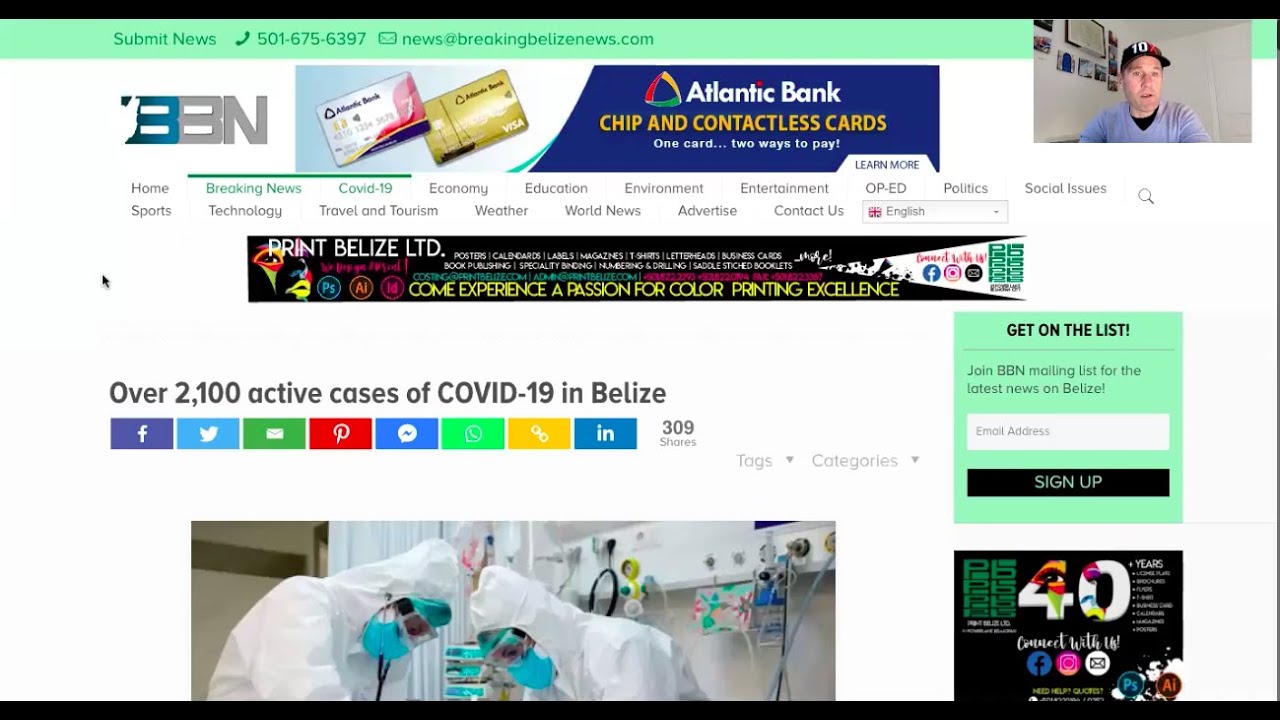The image showcases a screenshot of the BreakingBelizeNews.com (BBN) website. Positioned at the very top of the webpage are a "Submit News" link, a telephone contact number, and an email address (news@BreakingBelizeNews.com). The BBN logo is prominently displayed below this information, featuring a blue 'B' followed by grey 'B' and 'N,' all in uppercase letters. 

Adjacent to the BBN logo, an advertisement for Atlantic Bank promoting their chip and contactless cards is visible. An additional advertisement for Print Belize Limited is also present on the screen. In the top-right corner, there's an image of an individual wearing a baseball cap, presumably a key figure behind the website's operations.

Below the BBN logo and the Atlantic Bank ad, there is a navigation menu with headings that allow users to explore a variety of topics commonly found on news websites. These categories include Home, Breaking News, COVID, Economy, Education, Environment, Entertainment, Politics, Social Issues, Sports, Technology, Travel and Tourism, Weather, World News, Advertisements, and Contact Us.

The main splash screen prominently displays current information, noting that there are over 2,100 active cases of COVID-19 in Belize.